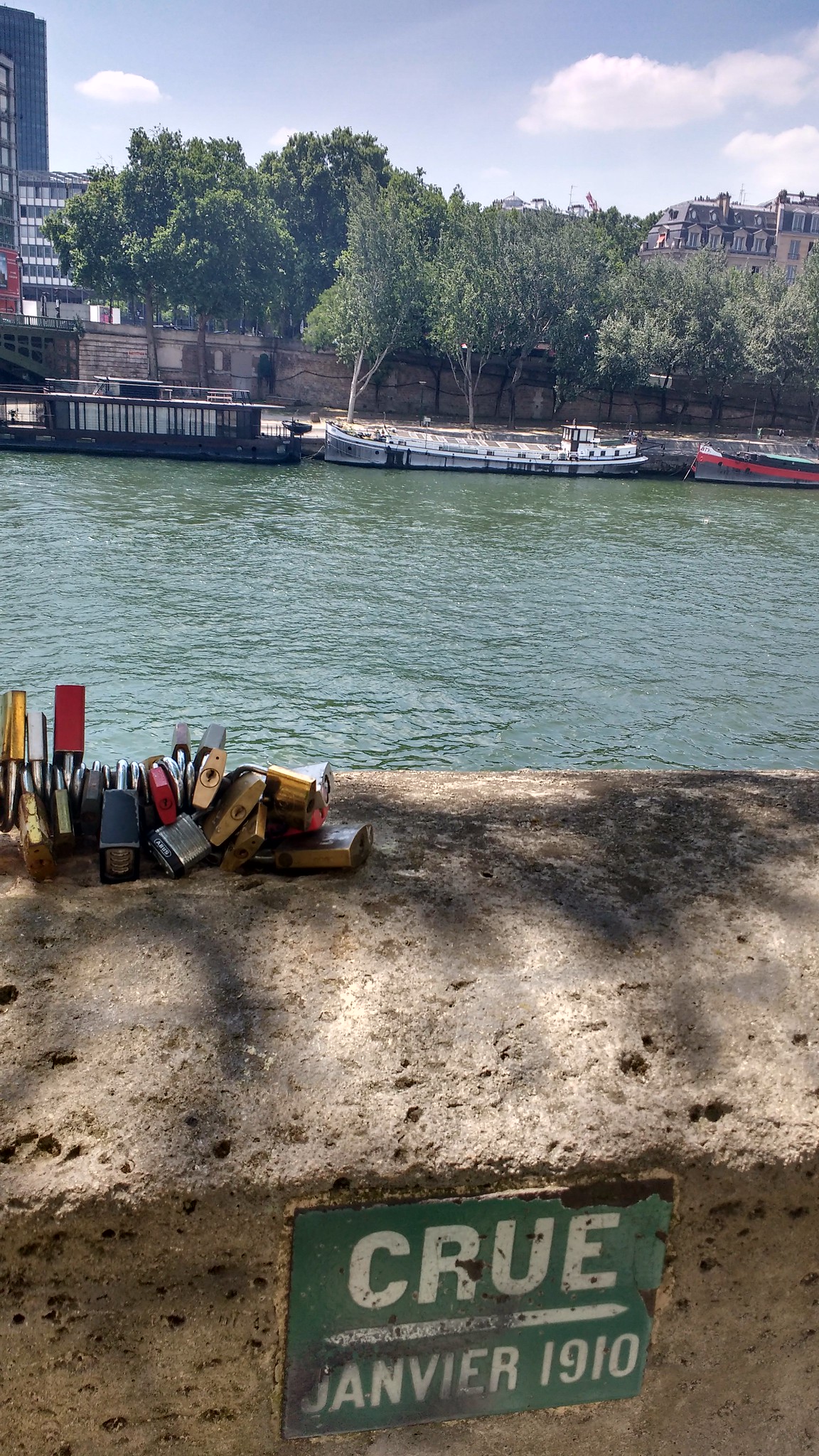The photo captures a tranquil urban river scene from an elevated vantage point on a bridge. In the foreground, a stone ledge or railing is adorned with numerous colorful padlocks, affixed to a metal bar that stretches from the center of the image off to the left. Attached to the stone railing, a small green sign with white letters reads, "Crew Jan Veer 1910," marking a point of historical interest. The water below is calm, with several flat boats moored along the far bank. Leafy deciduous trees create a natural barrier behind the boats, and beyond them, city buildings rise into the sky. The architecture is diverse, with modern skyscrapers clustering on the left and a more historic building featuring a mansard roof and multiple windows standing prominently on the right. The sky above is sunny with a scattering of clouds, casting a serene light over the entire scene.